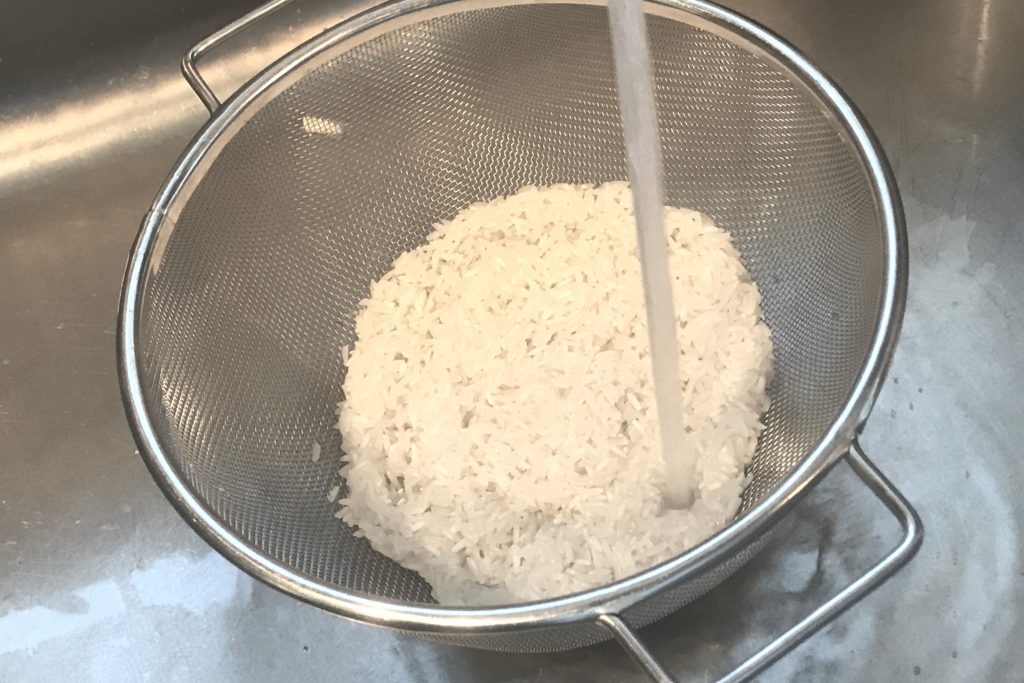This image depicts a top-down view of a stainless steel colander positioned inside a matching stainless steel sink. A thin stream of water from an unseen faucet is pouring directly into the colander, which contains a bed of white rice. The colander has a handle at both its front and back, suggesting ease of use for rinsing or shaking its contents. The rice appears to be uncooked and is being washed, as indicated by the water flowing over it. The metallic, shiny finish of both the colander and the sink is clearly visible, mirroring the typical appearance of kitchen appliances. Small specks of rice are also visible around the colander, reinforcing the action of washing the rice.